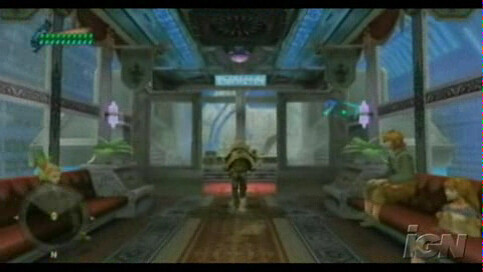This detailed screenshot appears to be from a video game, indicated by the transparent "IGN" watermark in the bottom right corner. The scene captures the interior of a possible waiting area or transport vehicle, with walls and doors made predominantly of glass framed in dark material, giving the space a modern, sleek appearance. 

In the foreground, there's a character facing away from the viewer, dressed in black and white armor or a black jacket and pants with a white stripe on the back. They seem to be heading towards a large glass doorway that emits a glowing red light in the middle of the room.

The setting also features a central rug with a distinct design: a blue border on the outside, followed by a tan border, and a thicker brown strip in the center. The rug runs down the middle of the floor, drawing the eye towards the glass doors beyond.

On either side of this central path are rows of red or reddish-maroon couches. To the left, a woman with light brown hair, wearing a gray and green sweater with brown capri pants, sits calmly. A few seats away from her is a child in a dress with light brown hair. Across the aisle, on the right, two more individuals are seated: one, a man in a greenish shirt and brown pants, and another, a woman in a white shirt and red skirt. Another child with blonde hair is among the seated individuals on the right side.

Additionally, the top left corner of the image displays a bar filled with green lights, possibly indicating health or progress status within the game. In the bottom left, a dark black compass with a gray outline points north, adding further to the interface elements typical of a video game. The ceiling above reflects a blue light, enhancing the futuristic atmosphere of the scene.